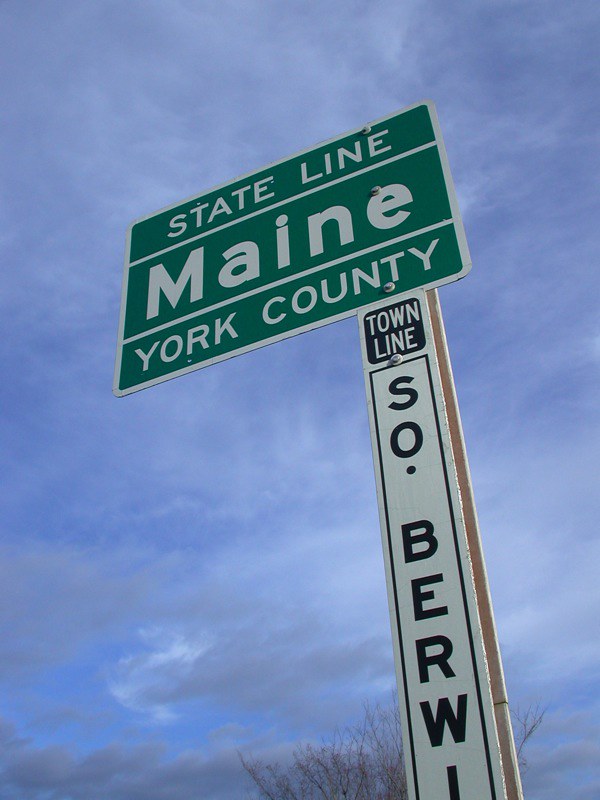A green street sign stands prominently against a clear blue sky, indicating the "State Line" for Maine and "York County." Below it, a white sign reads "Town Line," partially obscuring the name to "Burw" before it cuts off. The dead trees at the bottom of the image suggest it's winter, with the leafless branches adding a stark contrast to the vibrant sky. Wispy clouds float above, creating an intricate pattern that adds a dramatic touch to the scene. Besides the signs and trees, the image is dominated by the expanse of the sky, giving it an open and airy feel.